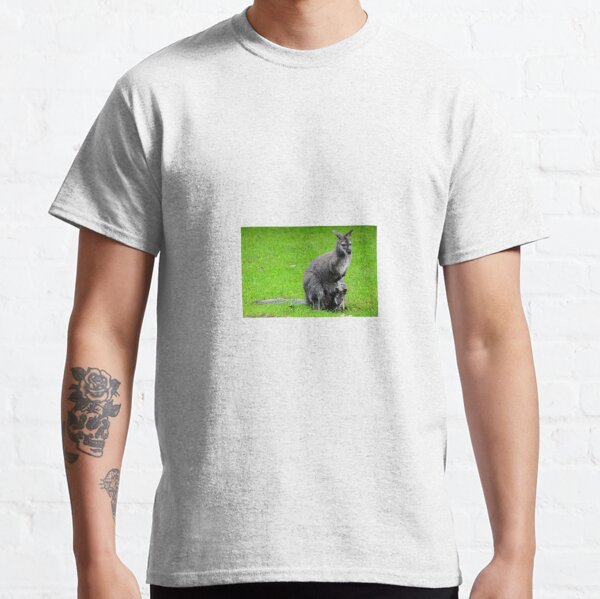In this image, a young male with fair skin is modeling a white short-sleeve t-shirt. The t-shirt features a centrally placed photograph of a kangaroo, which appears grayish-brown and is set against a bright green grassy field. The image on the shirt is somewhat small and unesthetically placed, making it appear a bit awkward. The man's face is cropped out of the image; you only see him from the neck to the waist. His left arm, resting at his side, showcases a tattoo of a skull with a rose on the bottom half, inked in a dark color. He stands against a white-painted brick wall, further highlighting the plainness of his attire.